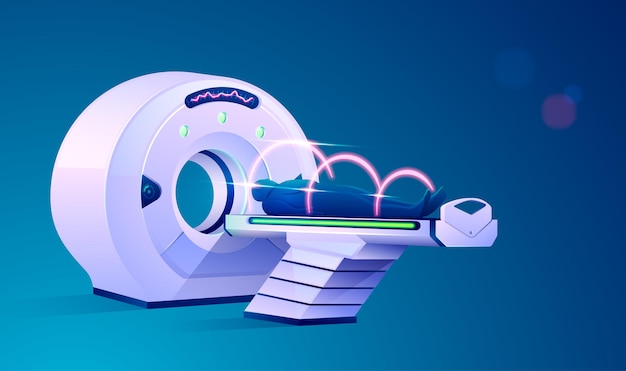This detailed digital art representation likely depicts a CT or MRI scan machine, placed against a gradient backdrop transitioning from dark blue to turquoise. The main machine, characterized by its large circular shape with a central opening, showcases a futuristic design comprising light gray, off-white, and blue hues. It features three prominent green lights surrounding the central hole. A patient, positioned head-first on a predominantly white table with blue trim and touches of green and gray, is about to be inserted into the scanning machine. The patient is encircled by three pink, dome-shaped areas, suggesting focal points for imaging. Additionally, three iridescent orbs float near the right side of the image, enhancing its advanced, technological aesthetic.